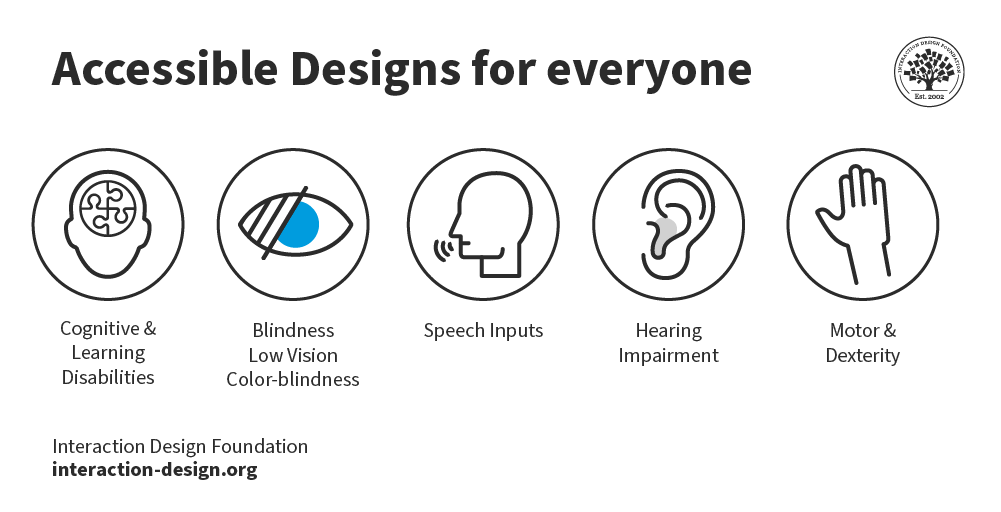The image is titled "Accessible Designs for Everyone" and features five distinct symbols representing different types of disabilities. The first symbol addresses cognitive and learning disabilities, depicted as a silhouette of a human head with puzzle pieces inside to represent the brain. The second symbol represents blindness, low vision, and colorblindness, illustrated by an eye with a blue pupil and two black diagonal lines crossing over it. The third symbol focuses on speech inputs, showcasing a human head with sound waves emanating from the mouth. The fourth symbol denotes hearing impairment, illustrated by a close-up of an ear. The fifth and final symbol stands for motor and dexterity issues, represented by a hand. Each symbol is enclosed in a circle and appears above corresponding text labels. The design is black and white, with a logo resembling a tree in the top right corner, which appears to be related to the Interaction Design Foundation's website, interaction-design.org.